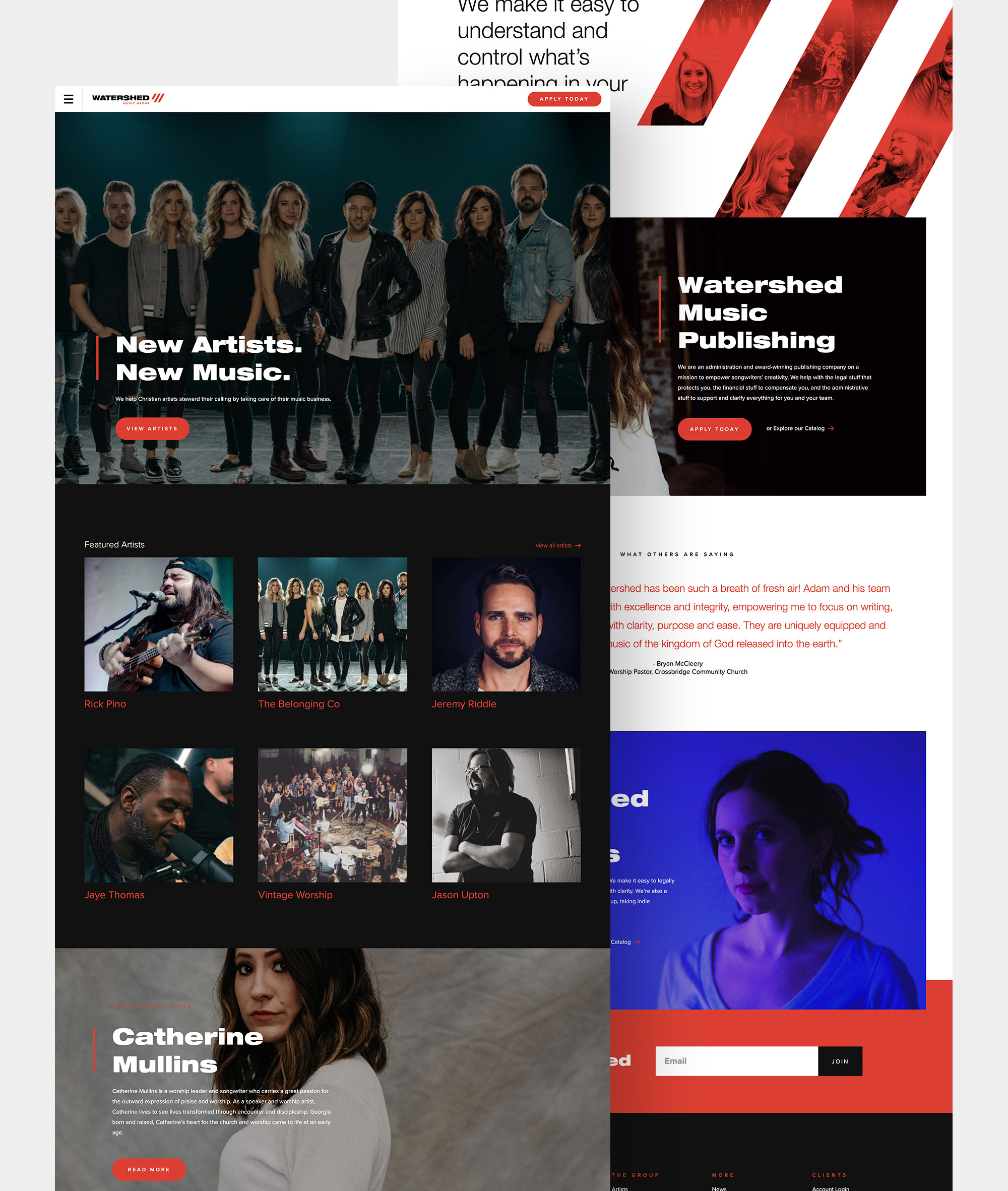The image displayed on the application webpage is divided into two primary sections: foreground and background. In the foreground, positioned slightly to the left, is a highlighted section labeled "Way Up Water: Watershed." This section announces "New Music, New Artists" and invites users to "View Artist" and "Apply Today." The text has a distinctive gradient effect, blending into a vibrant red background.

Occupying the top right of the image, the word "Origin" subtly overlaps the main elements. Prominently featured in the foreground are several individuals, presumably musicians, characterized by their distinct styles, who are facing forward.

The lower part of the foreground highlights "Featured Artists," listing names such as Rick Pino, The Belonging Co., Jeremy Riddle, Jason Upton, Vintage Worship, and J. Thomas, along with Catherine Mullins. Additionally, partial background text suggests an approachable and understandable control over the platform with the phrase "We make it easy to understand and control what's happening in you," though some words are obscured by the foreground.

On the right side of the background, visible text reads "Watershed Music Publishing - Apply Today." The webpage, identifiable as a music publishing site called "Watershed Music Publishing," integrates a black background interspersed with red elements. Furthermore, there is a search bar, and in the bottom right corner, an email input field encourages users to subscribe, underlined by a red background.